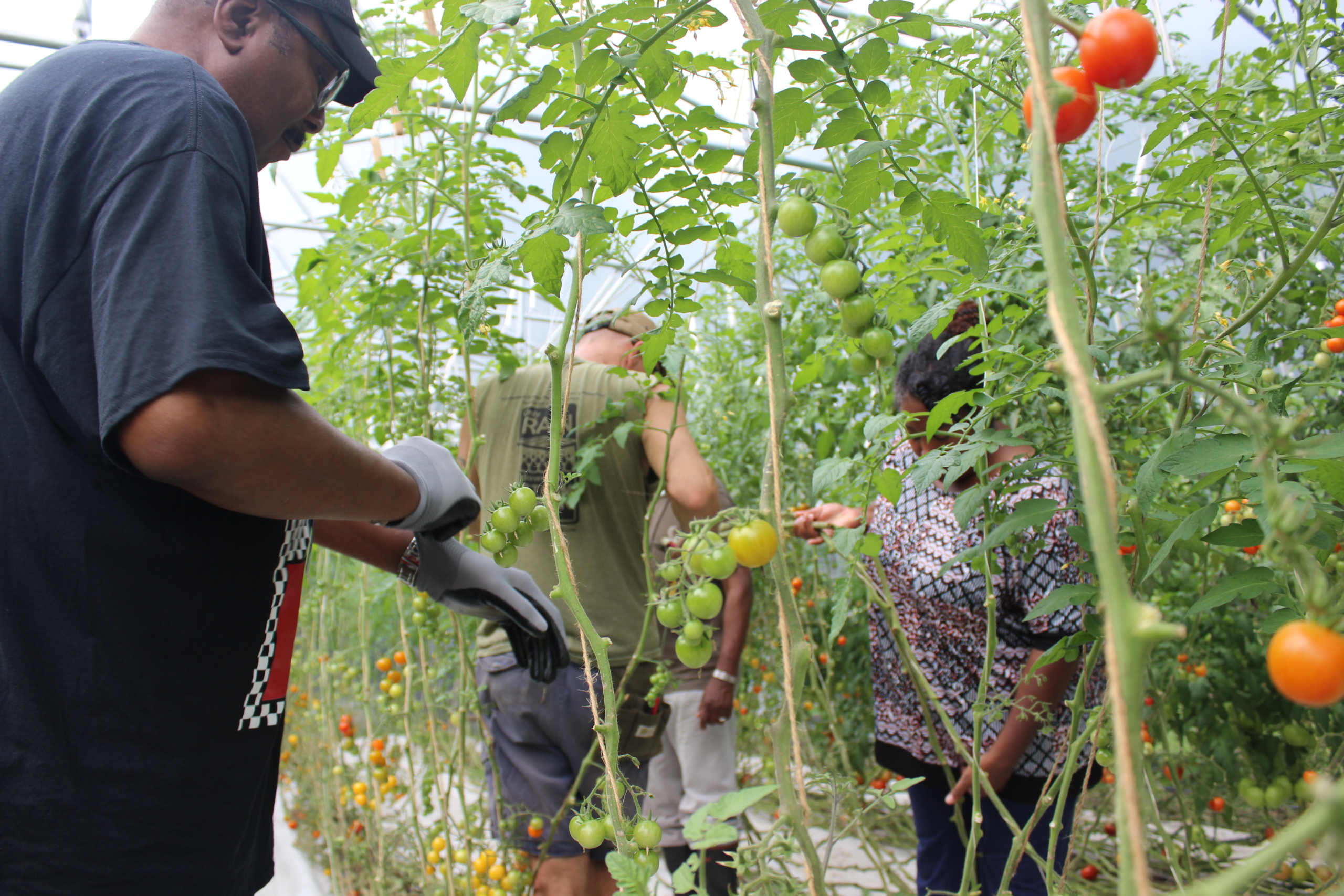In this detailed photorealistic image, taken from a knee-height perspective, we observe a community working together in a thriving tomato garden. Captured during the day under a partly cloudy sky, the lush vegetation includes towering tomato plants, some reaching up to eight feet tall. The tomato plants are laden with fruits in various stages of ripeness, from green and yellow to orange and vibrant red.

Among the tall vines, four individuals are engaged in picking and inspecting the tomatoes. On the lower left, a darker-skinned individual with potential Mexican heritage faces three o'clock, busy with a great box. Central to the scene is a darker-skinned male, likely of African American descent, wearing a green muscle shirt and tending to the plants. Just to the right stands a woman with brown hair in a purple-patterned shirt, also appearing to be of Mexican heritage, focused on her task.

Additionally, a partially obscured person in the background adds to the sense of a bustling, cooperative effort in the garden. The collective activity illustrates a shared commitment to cultivating this community garden, reflecting a harmonious blend of ethnicities and a shared purpose amidst the lush, productive setting.